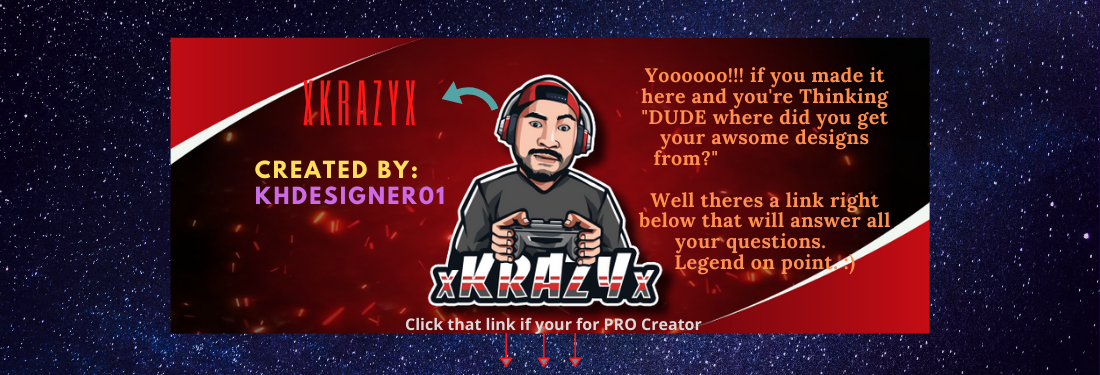This promotional banner advertisement encourages people to connect with the designer for their business needs. The horizontal rectangle features two red fields with white stripes in the upper left and lower right corners. Centered between these frames is a cartoon-colored pencil depiction of an Asian gamer, presumably a streamer, wearing headphones, with a mustache and beard, dressed in a gray long-sleeve shirt with white shoulder stripes. He appears to be holding a game controller.

Above his head, an arrow points to the left, directing attention to his screen name, "XKRAZYX," written in red lettering on a dark red background. Below this, in yellow text, the words "Created by:" lead to "KHDesigner01" written in purple on the same dark red background.

To the right of the cartoon figure, in gold or yellow text over the dark red background, are two paragraphs: 
- "Yahoo!!! If you made it here, you are thinking, 'Dude, where did you get your awesome designs from?'"
- "Well, there's a link right below that will answer all your questions. Legend on point. :-)"

Directly below the cartoon, in outlined white text, is "XKRAZYX," and under that, in white lettering on the red background, with three red arrows pointing downward, it reads, "Click that link if you're for Pro Creator."

While the advertisement features high-quality graphics, it shows signs of amateur construction due to misspellings and formatting issues. Nonetheless, it is a reasonably crafted piece that could benefit from some editing.